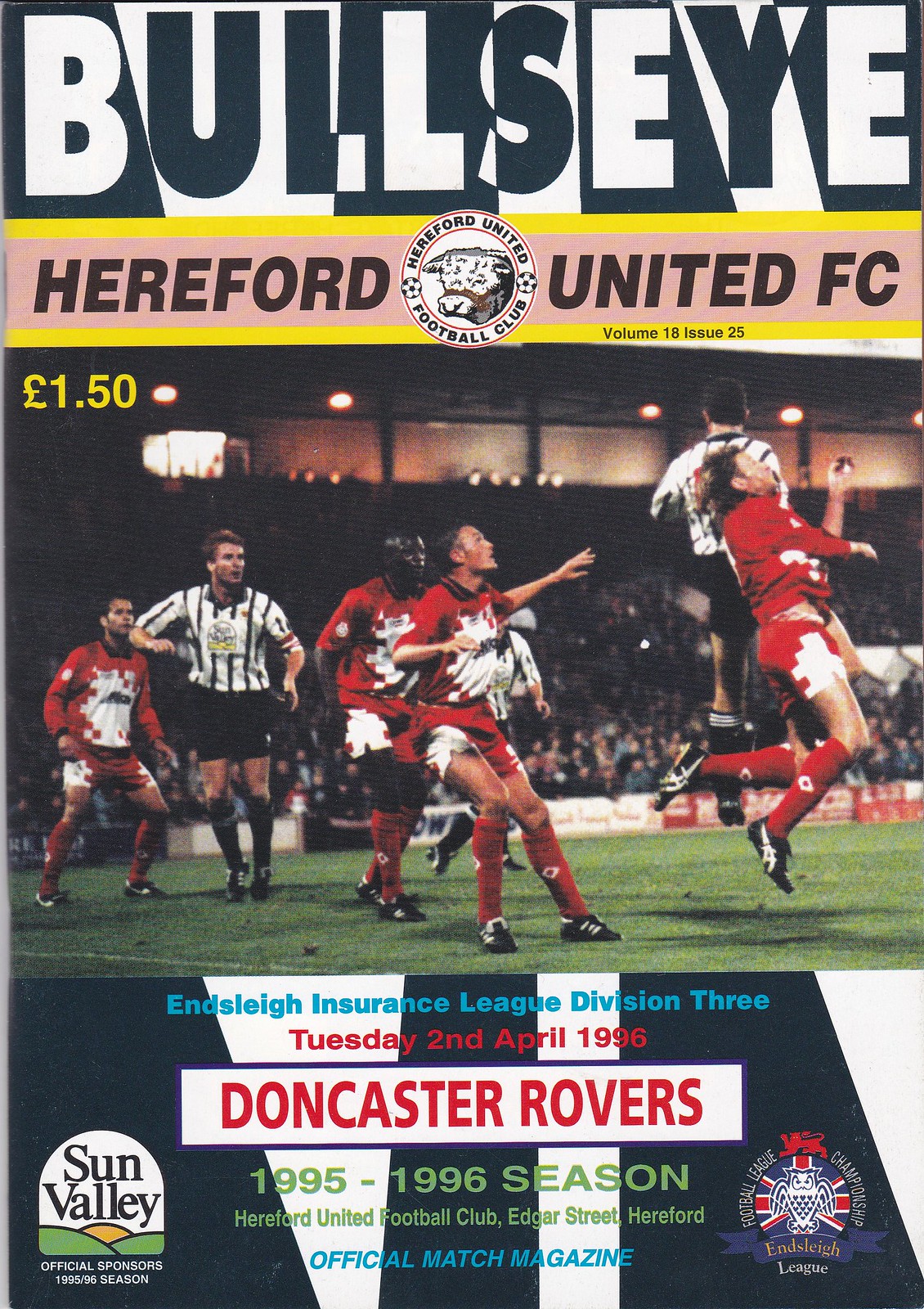The cover of this magazine, titled "Bullseye," prominently features the Hereford United FC women's soccer team in action, donned in red and white uniforms with matching red socks. The title "Hereford United FC" is boldly set in black letters at the top against a black and white background. Below it, a dynamic photograph captures the players and a referee, who is dressed in a black and white striped shirt with black shorts, in the midst of a game on a green field with white lines. Surrounding the photo is a contrasting design: a pink backdrop outlined in yellow containing the price of £1.50 in yellow font and various team symbols.

The bottom section presents key details in black and white, with crucial information in blue and red. It announces the Enslay Insurance League Division III match, scheduled for Tuesday, April 2, 1996, featuring the Doncaster Rovers and Hereford United FC for the 1995 to 1996 season. Additional adornments include advertisements, such as one from Sun Valley in the bottom left corner featuring a logo with green hills and a yellow sun, labeled as the "Official Sponsors." The right corner hosts another emblem with "Enslay" in yellow on a purple ribbon. All these elements, set on a black background with white and red lettering, make for a vibrant and informative cover highlighting the sportsmanship and season details of the Hereford United Football Club.